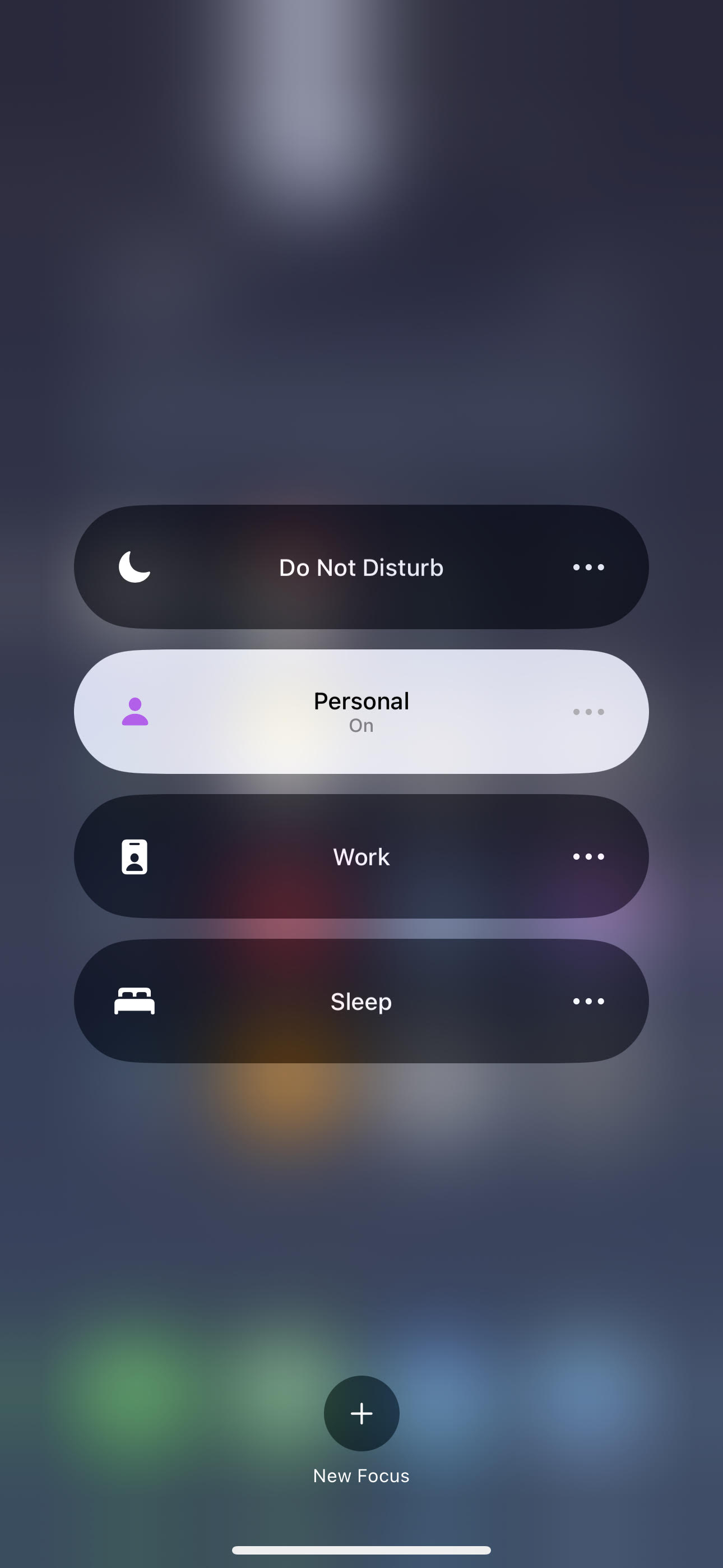The image displays a smartphone screen with a slightly blurred background featuring a typical home screen layout. Prominently shown are four distinct focus mode options with corresponding icons and dropdown menus: 

1. **Do Not Disturb**: Represented by a moon icon, this option helps to mute notifications.
2. **Personal**: Illustrated by a white person icon, it indicates the phone’s personal mode, with a dropdown menu beside it.
3. **Work**: Marked with an icon resembling a badge, designated for work mode, also featuring a dropdown menu within a black box.
4. **Sleep**: Depicted by a bed icon, used to manage settings during sleep, accompanied by a dropdown menu.

At the bottom, there is a plus sign followed by the text "New Focus," suggesting the addition of a new focus mode. The center of the screen features a white bar, centered horizontally, while background icons are softly masked by a muted blue overlay, adding a subtle contrast to the overall aesthetic.